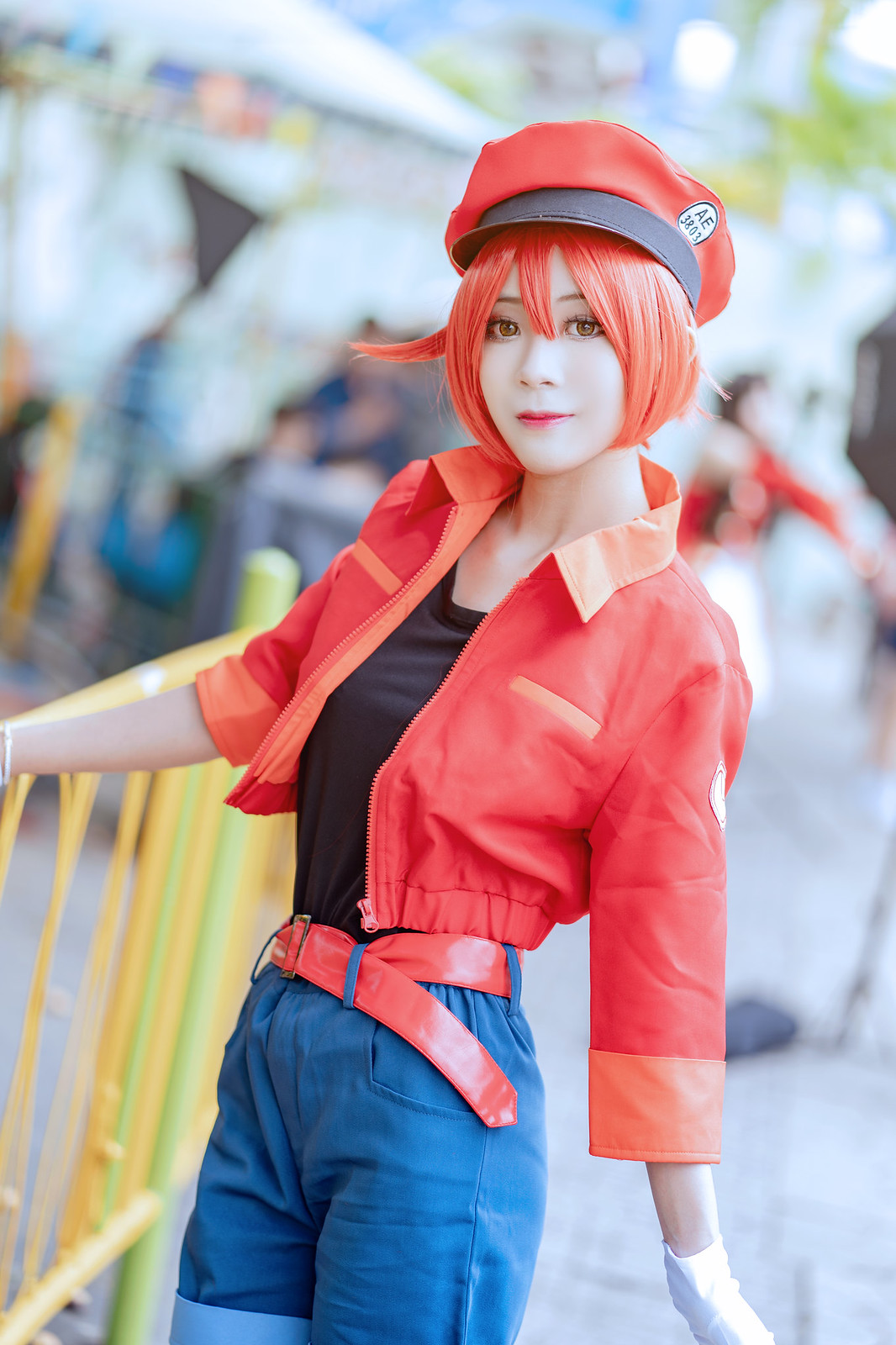In this vertical rectangular, full-color photograph taken outdoors during the daytime, a young woman—possibly in her twenties—is captured in an artistic, model-like pose. Her strikingly pale complexion and vibrant orange hair immediately draw attention. She wears an orange hat adorned with a black band, and her eyebrows, eyes, nose, and mouth are clearly visible. Her outfit consists of an orange jacket layered over a black tank top, denim shorts cinched with an orange belt, and a glove on one visible hand. The woman is holding onto a thin yellow railing with the gloved hand while leaning back slightly, giving the impression that her weight is supported by the railing. The entire background is blurred and abstract, yet it suggests an outdoor setting, possibly with elements resembling a merry-go-round. The overall composition of the photograph emphasizes both the vivid colors of her attire and her poised stance.